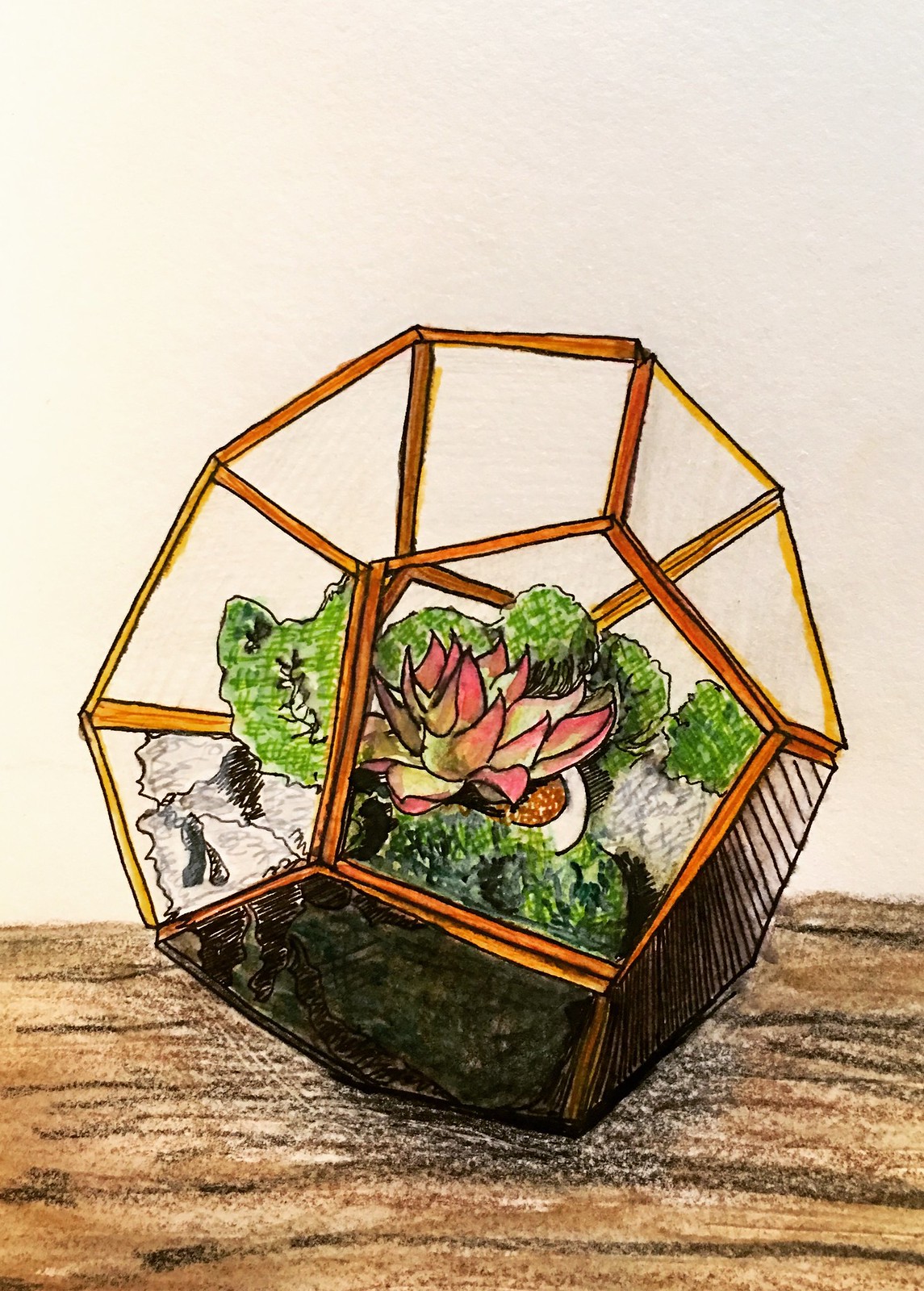This detailed artwork depicts a hand-drawn, hexagonal glass terrarium filled with a miniature garden of plants. The illustration, likely created using crayons, colored pencils, and possibly a black fine line marker, features a distinct brassy skeletal frame colored in hues of orange and gold. The transparent glass panes of the terrarium reveal a rich, dark brown layer of soil along with assorted light gray rocks. A variety of green plants thrive inside, with a prominent, spiky red or pink-tipped succulent plant serving as the central focal point. This intricate terrarium artwork rests on a wooden tabletop, rendered in brown crayon, emphasizing the natural and earthy theme of the composition.